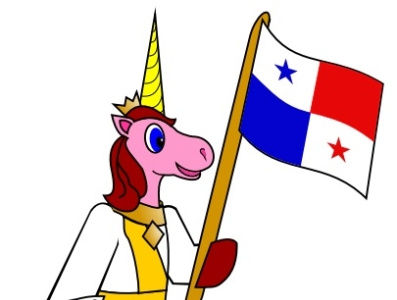The image is a whimsical, cartoon drawing of a unicorn seen from its right side. The unicorn has a pink face with blue eyes and is adorned with a small yellow crown and a yellow horn. It has red, shoulder-length hair and a red left hand that holds up a flag with a yellow rod. The unicorn is dressed in a white jacket over a yellow shirt. The flag is divided into four quadrants: the top left and bottom right are white with a blue star in the top left and a red star in the bottom right; the top right quadrant is red, and the bottom left quadrant is blue. The enchanting style of the image, with its vibrant colors and fantastical elements, suggests it could be from a children's book.